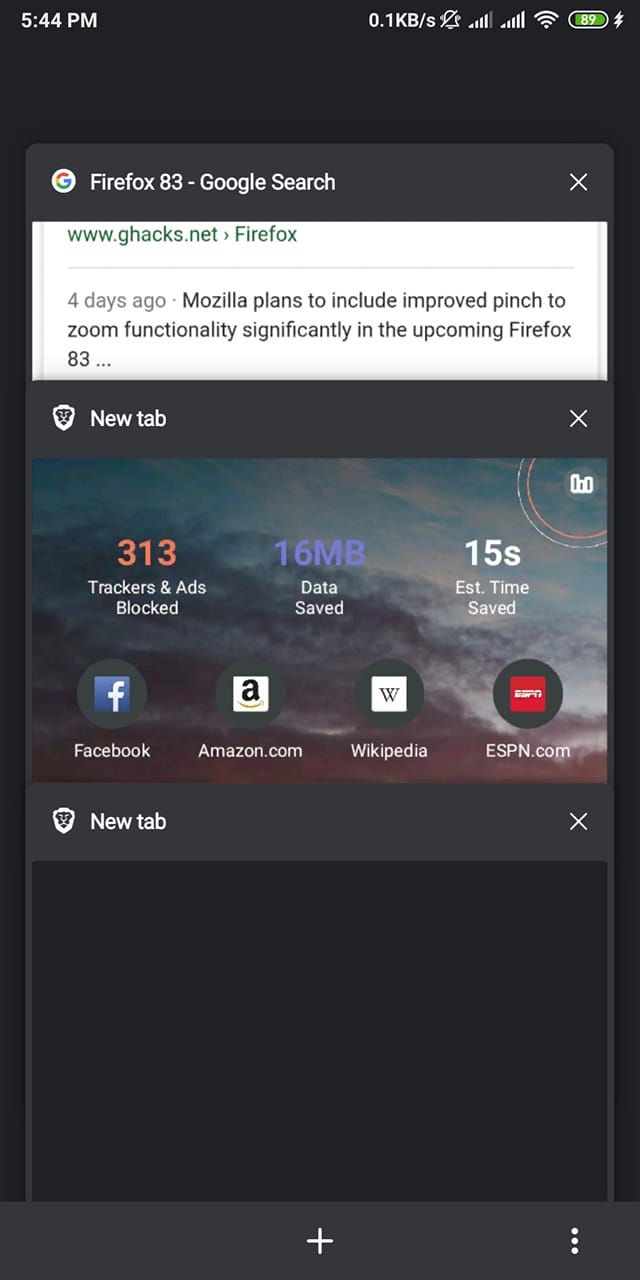This is a screenshot taken from a smartphone. The majority of the background is black. In the top left-hand corner, the time is displayed as 5:44 p.m., and the battery level is indicated at 89% with a charging symbol and a green progress bar. The web browser in use is Firefox, showing the tab "Firefox 83 - Google Search," and a colorful Google "G" icon is present.

The URL displayed is www.ghacks.net, and the page headline reads, "Mozilla plans to include improved pinch-to-zoom functionality significantly in the upcoming Firefox 83..." with the rest of the headline truncated. An option to open a new tab is visible.

In the middle section of the screen is a graphic resembling a beautiful sky. Below this graphic, statistics are shown: "313 trackers and ads blocked," "16 MB data saved," and "15s estimated time saved." Additionally, there are icons for Facebook, Amazon.com, Wikipedia, and ESPN.